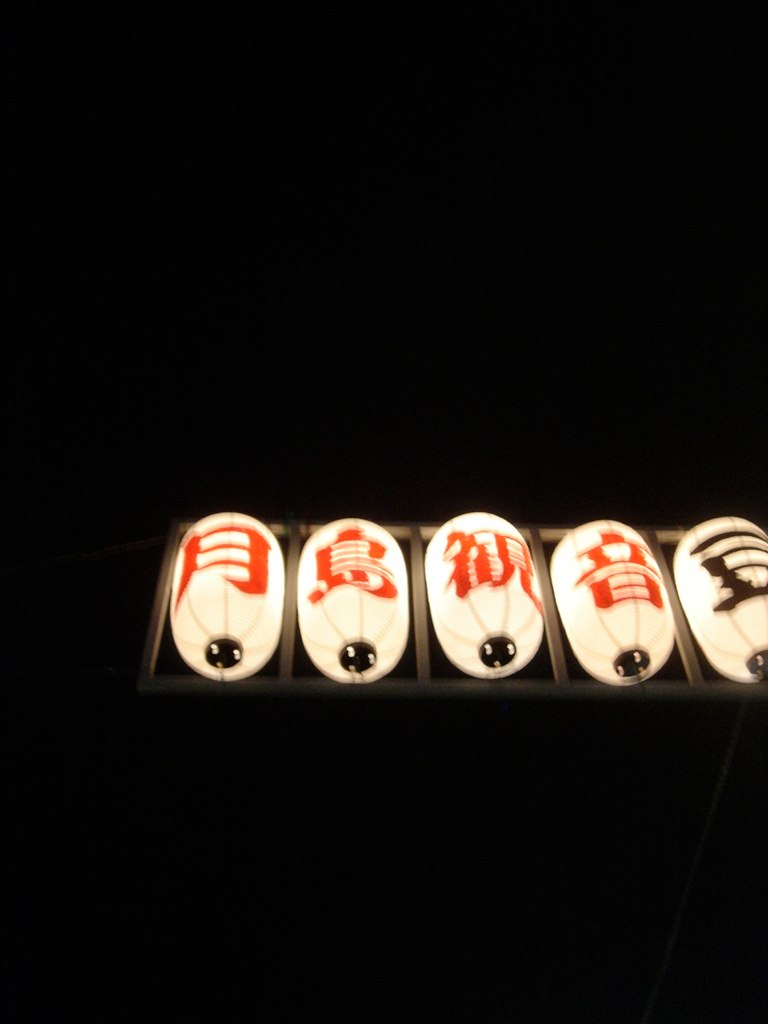In this image, set against a backdrop of an impenetrably dark night sky devoid of stars and the moon, a lit-up sign is the sole source of illumination. The sign, consisting of five horizontally aligned lanterns, is suspended on metal rods. The lanterns are shaped in an oblong, roundish form with a resemblance to paper material, exuding a warm white light that shines through their framework. Each lantern features inscriptions in Japanese or potentially another Asian script: the first four exhibit characters in bold red, while the fifth, positioned on the far right, showcases black lettering. All lanterns are designed with a black plastic base. The image captures a blend of traditional aesthetics and modernity, evoking the charm of old-fashioned lanterns which would have been candlelit in the past but are now electrically powered. The stark contrast between the bright lanterns and the pitch-black sky creates a striking and evocative scene.